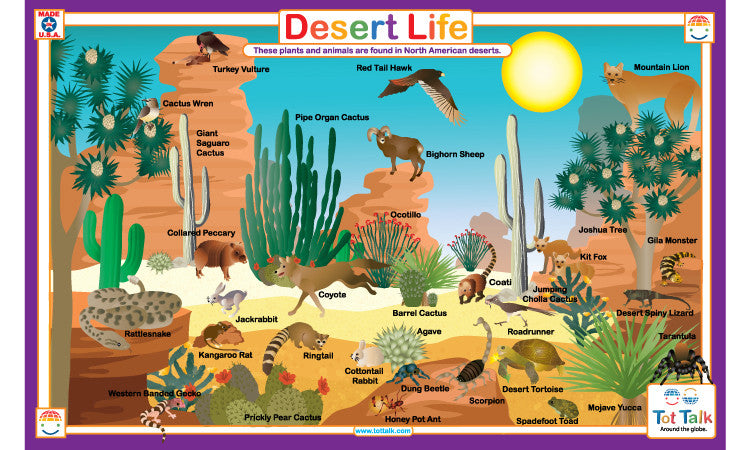This is an illustration from a book titled "Desert Life," framed with a thin purple border and an inner white frame featuring various logos at the corners. In the top left, a blue circle with a white star says "Made in the USA." The top right and bottom left corners display a smiley face with a red and orange globe as the top half of the head, while the bottom right features the same smiley face, one upright and one inverted, with the words "Taut Talk" around the globe. At the top center, a white rectangle with rainbow-colored lettering spells out "Desert Life," and below it, a white lozenge states, "These plants and animals are found in North American deserts."

The scene depicts a vivid desert landscape with rocky outcroppings, various cacti, and desert plants against a turquoise sky with a yellow sun bordered in orange. There are flowers, sagebrush, sandy terrain, and differing sand colors indicating shadows and sunlight. Scattered across the scene are multiple desert animals and plants, including a turkey vulture, cactus wren, giant saguaro cactus, collared peccary, rattlesnake, jackrabbit, kangaroo rat, Western banded gecko, prickly pear cactus, ringtail, coyote, pipe organ cactus, red-tailed hawk, bighorn sheep, ocotillo, barrel cactus, agave, cottontail rabbit, dung beetle, honeypot ant, scorpion, spadefoot toad, Mojave yucca, desert tortoise, tarantula, desert spiny lizard, roadrunner, coati, jumping cholla cactus, kit fox, Gila monster, Joshua tree, and mountain lion. Each plant and animal is labeled in small black text, enhancing the educational aspect of the illustration. The flat colors with deep shading give the artwork a unique blend of cartoonish and realistic elements.